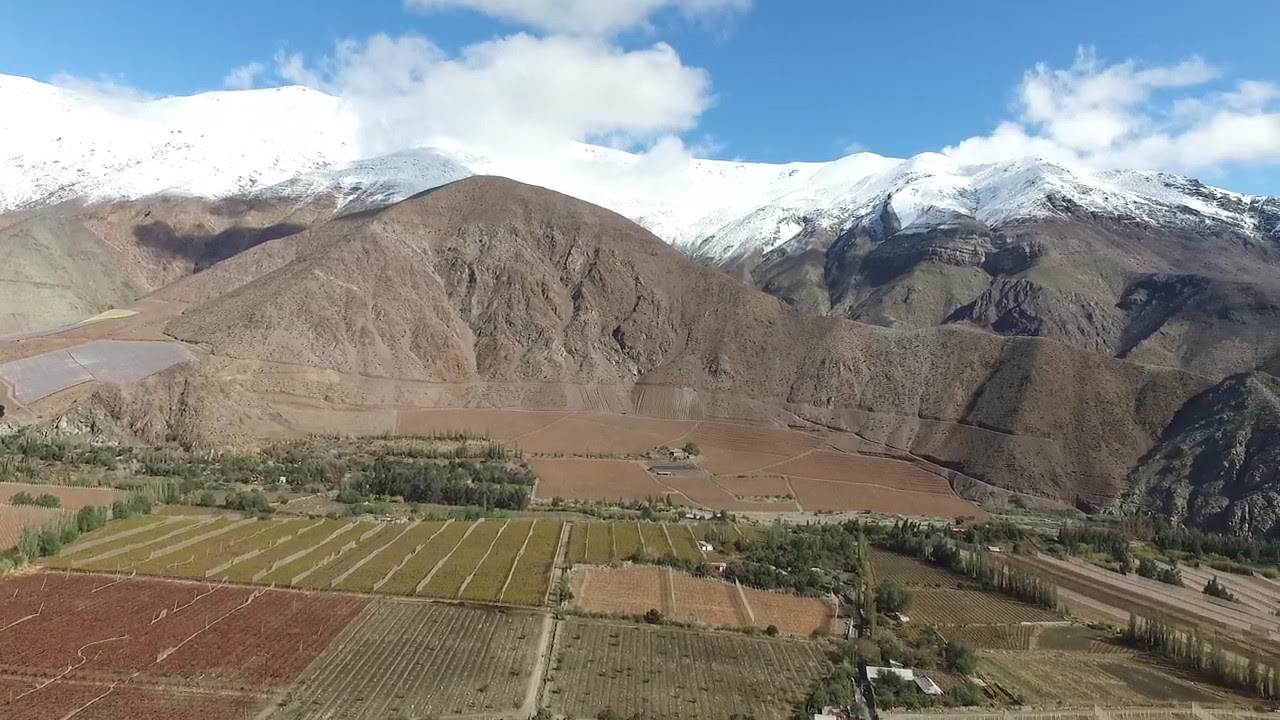This stunning aerial photograph captures a picturesque valley scene where cultivated fields stretch across the lower third of the image. These fields, varying in shades of brown and gray, show distinct rows and appear to be either plowed or planted. The fields are bordered by windbreaks of trees, and a road weaves through the right side of the picture, further enhancing the orderly agricultural landscape.

In the middle of the composition, the terrain begins to rise into a series of foothills, characterized by their solid brown color and sparse vegetation. As the eye travels further back, the terrain transitions into a magnificent mountain range that spans the entire width of the image. These mountains exhibit a soft light gray hue, with some jagged peaks adding texture to their smooth surfaces.

The farthest mountains, particularly those on the left and right sides of the image, are crowned with gleaming white snow, signifying their higher elevations. Above this stunning landscape, the sky stands out with its vibrant blue color, dotted with a few fair-weather clouds scattered mostly towards the right and left middle side of the scene. The overall composition beautifully contrasts the cultivated fields, barren foothills, and the majestic, snow-capped mountains under a serene blue sky.